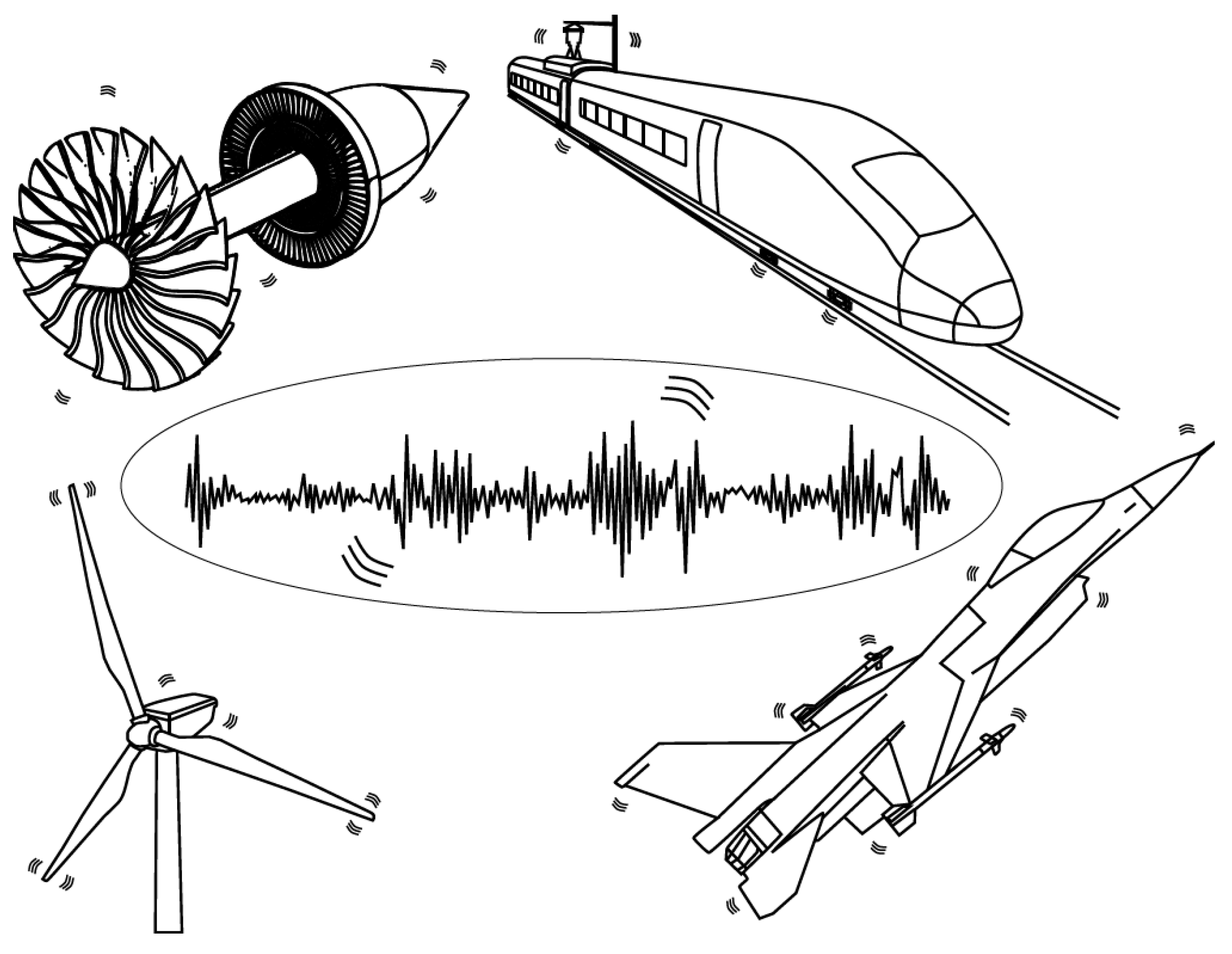This black-and-white sketch, resembling pencil art on a white background, intricately depicts various objects related to thrust and motion. In the center, a long oval shape features dynamic sound waves, reminiscent of vocal sound patterns. Encircling this central motif, in a clockwise direction, are distinct illustrations: the upper left shows a bladed propeller with a conical attachment; the upper right displays a sleek commuter train with a sloped nose, resembling a monorail or subway train, complete with a visible front car and a following car. The bottom right captures a fighter jet equipped with two missiles, while the bottom left portrays a segmented wind turbine. Each object is augmented with subtle action lines, hinting at motion or vibration, adding to the dynamic nature of the composition.